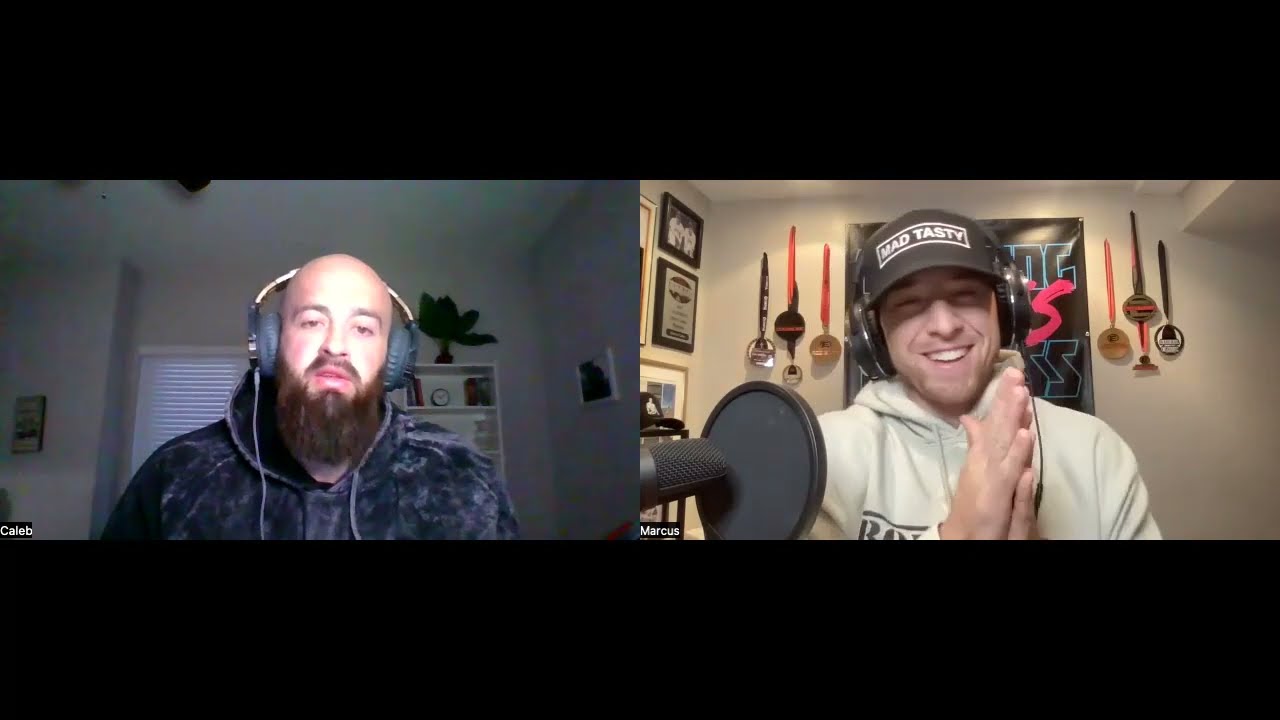The image is a screenshot of what appears to be a podcast recording featuring two men captured via their webcams. Both men are shown from the chest up, wearing headsets and seated in their respective rooms.

On the left, Caleb, a bald man with a brown beard, is dressed in a dark blue and gray felt-textured hoodie. His room has plain white walls, and in the background is a white bookshelf with a plant on top and white window shades. He wears large gray headphones with a visible cord on the left side.

On the right, Marcus, wearing a cream-colored hoodie, a black cap with "MAD TASTY" written on it in white font, flashes a toothy smile, revealing his clean, straight, white teeth. His background includes several medals, framed diplomas, and awards mounted on the white walls, along with a large black poster. Marcus is positioned in front of a black microphone, adding to the podcast setting ambiance.

Both settings appear to be well-lit, contributing to the clear and bright quality of the image.